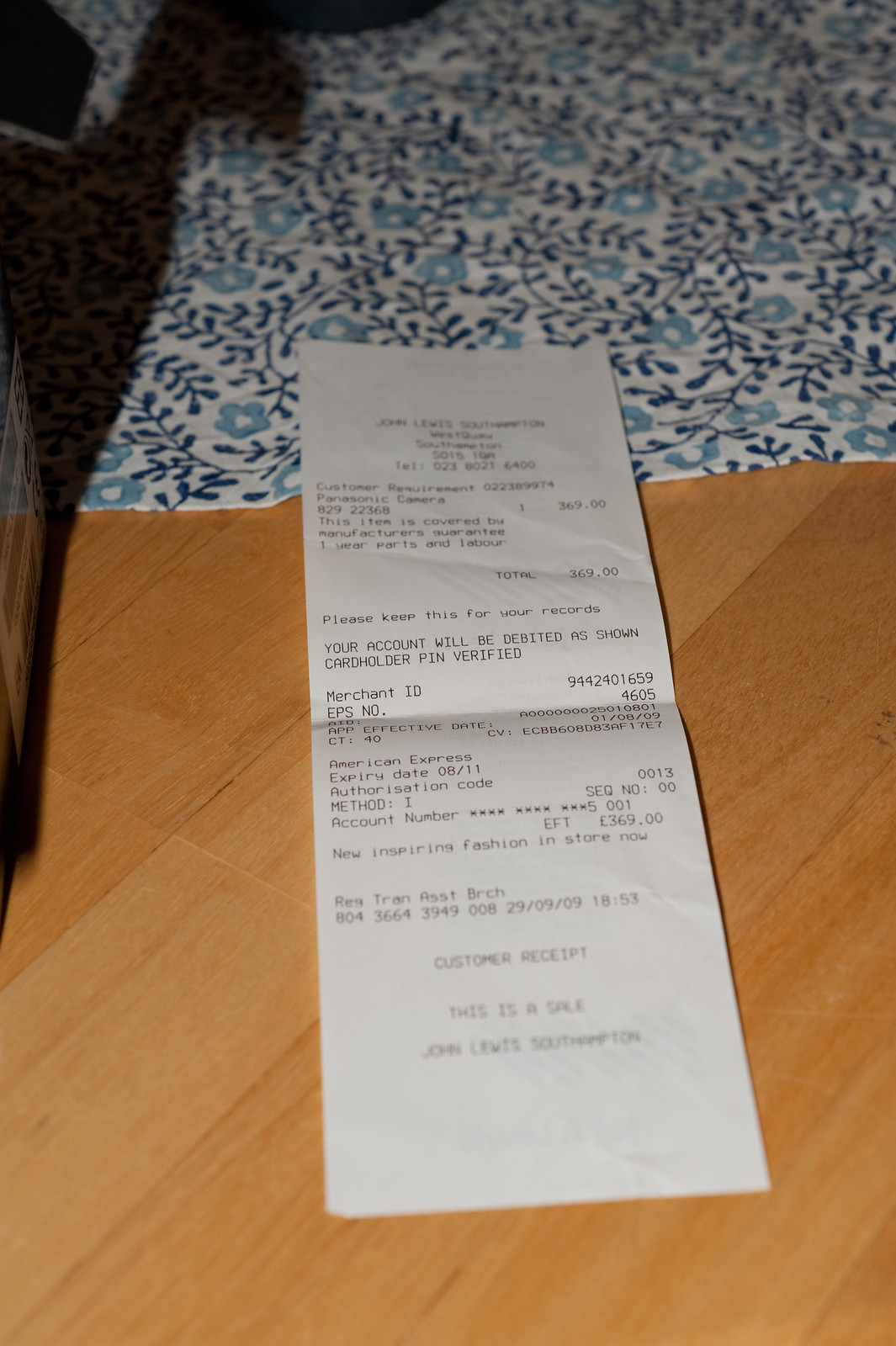A neatly printed receipt in black font is captured in this photograph. The receipt is laid partially on a blonde wooden table with visible gray wood grain, while the other half rests on a piece of fabric. This fabric features a white background adorned with blue leaves and smaller light blue flowers. Although the image is taken from a distance, making the text on the receipt difficult to decipher, the words "merchant ID" followed by a string of numbers and "customer receipt" at the very bottom are legible. Gentle reflections of light can be seen on the wooden surface, adding a touch of depth to the scene.